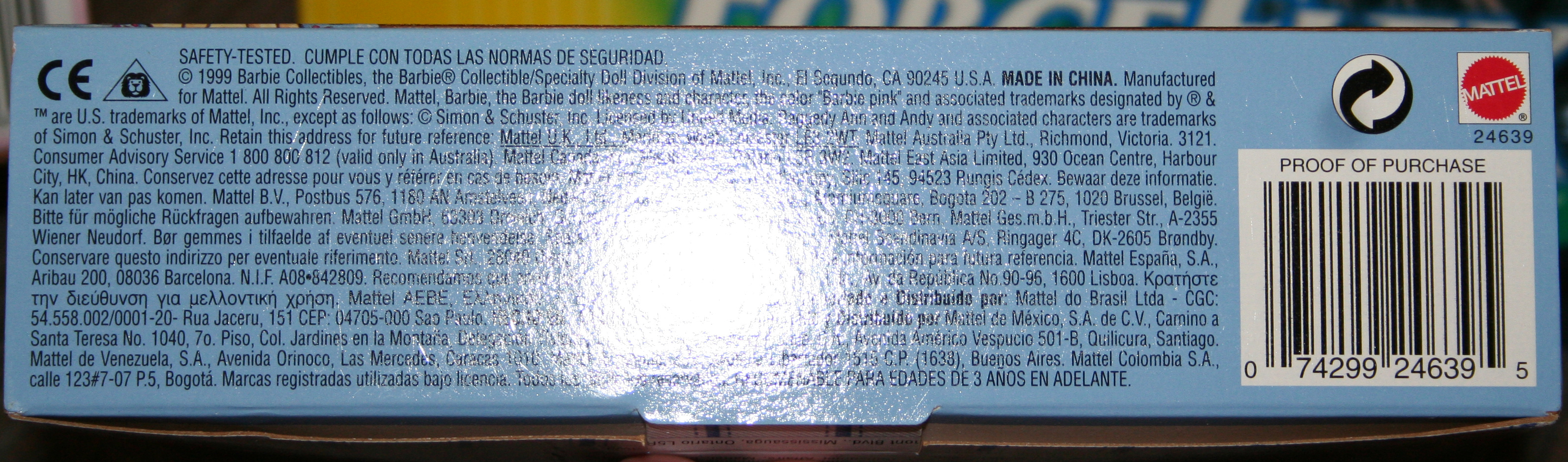The image portrays the bottom of a narrow, rectangular toy package. Central to the photo is a prominent circular reflection of light, creating a bright spot right in the middle. On the bottom right, a large barcode is present with the text "Proof of Purchase" displayed above it in black font. In the top right corner of the box is the red Mattel logo, a circular emblem with "Mattel" written in white, angled text. Next to the Mattel logo, there is another circle featuring two arrows, one black pointing right and one white pointing left. On the left side of the box, a CE logo is visible, followed by a triangle. The bottom of the box includes manufacturing details, safety test information, and additional multilingual notices.